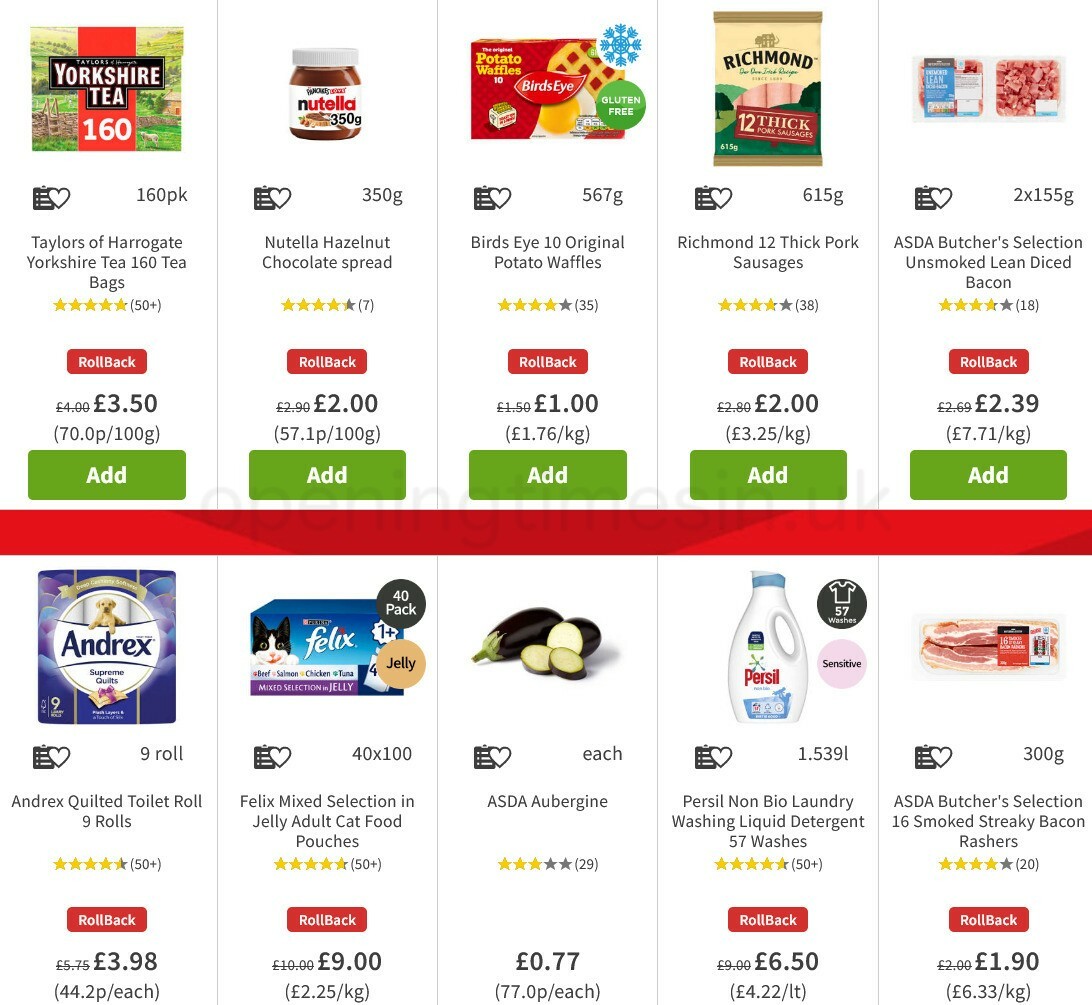A detailed panorama showcases a variety of food items from what appears to be either a single supermarket such as Kroger or Walmart, or an aggregator like Instacart. 

At the top, there's a box of **Yorkshire Tea** with 160 tea bags. The box features a picturesque farm scene and a clipboard with a heart symbol indicative of a favorite for later ordering. The text on the box reads "Tailors of Harrogate, Yorkshire Tea, 160 tea bags," with over 50 reviews and a perfect 5 out of 5 rating. A red rectangle with white text displays "Rollback." The original price of £4 is crossed out and discounted to £3.50, equating to 70 pence per 100 grams. A forest green "Add" button is also present.

Next to it is a jar of **Nutella Hazelnut Chocolate Spread** weighing 350 grams, rated 4.25 out of 5 stars. Initially priced at £2.90, it's now marked down to £2, which is 57.1 pence per 100 grams.

The third item is **Birdseye 10 Original Potato Waffles** at 567 grams, rated 4 out of 5 stars. Originally £1.50, it's reduced to £1, or £1.76 per kilogram.

Following this, there is a pack of **Richmond 12 Thick Pork Sausages**. Scoring 3.9 out of 5 stars from 38 reviews, it’s on sale for £2, reduced from £2.80, calculated as £3.25 per kilogram.

A pack of **ASDA Butcher Selection Unsoked Lean Diced Bacon** comes next, rated 3.8 out of 5 stars from 18 reviews. Previously priced at £2.69, it is now £2.39, amounting to £7.71 per kilogram.

An essential household item, **Andrex Quilted Toilet Roll** with 9 rolls, is rated 4.5 out of 5 stars from 50 reviews. Originally £5.75, it is now reduced to £3.98, which is 44.2 pence per roll.

A box of **Felix Mixed Selection in Jelly Adult Cat Food Pouches** with a black circle indicating a 40-pack and a brown circle for the "jelly" is next. Rated 5.7 out of 5 stars, possibly 8, it has been discounted from 10 euros to 5 euros, equating to £2.25 per kilogram.

A vegetable, **ASDA Egplant**, with a green stem and purple body is displayed. Rated 3 out of 5 stars from 29 reviews, it's marked at 77 pence, indicating 77 pence per eggplant.

**Personal Non-Binary Laundry Washing Liquid Detergent** for 37 washes has a rating of 4.8 out of 5 stars. A circular silhouette of a shirt with "57 washes" and textual elements indicating its sensitivity is featured prominently. It holds over 50 reviews.

Lastly, **ASDA Butcher Selection 16 Smoked Streaky Bacon Rashers** is displayed with a 4 out of 5-star rating from 20 reviews. Initially priced at £2, it's now £1.90, which translates to £6.33 per kilogram.